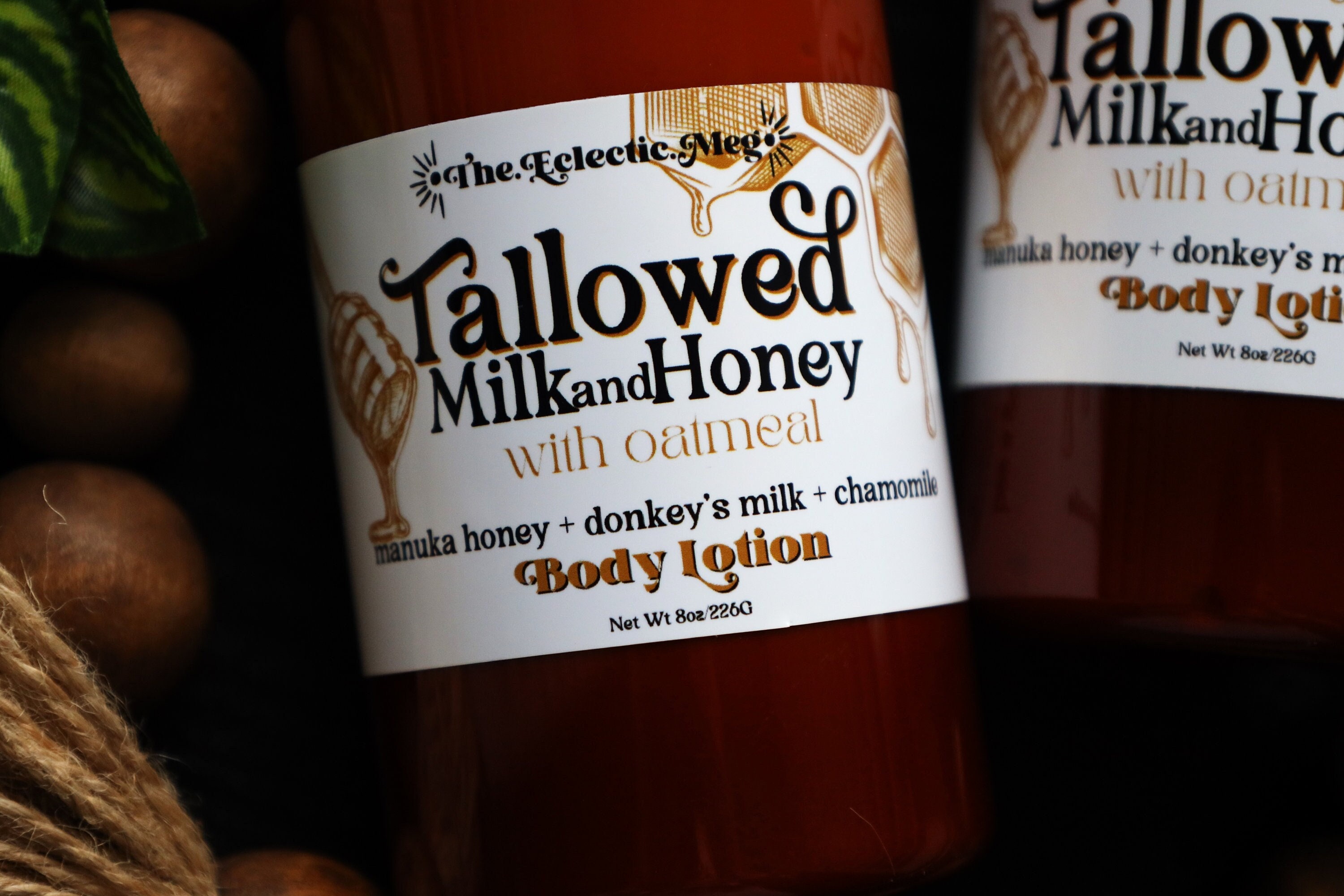This detailed promotional product photo by The Eclectic Meg showcases their "Tallowed Milk and Honey with Oatmeal" body lotion, featuring rich ingredients like Manuka honey, donkey's milk, and chamomile. The primary focus is on a brown, 8-ounce (226 grams) bottle with a white label and brown text displaying the product's name and main ingredients. The label also depicts a honey stick dripping with honey. To the right of the central bottle is a slightly cropped, identical bottle. To the left are various natural elements, including fruits like watermelon, potatoes, and strands of hemp cord, emphasizing the lotion's wholesome and natural components.